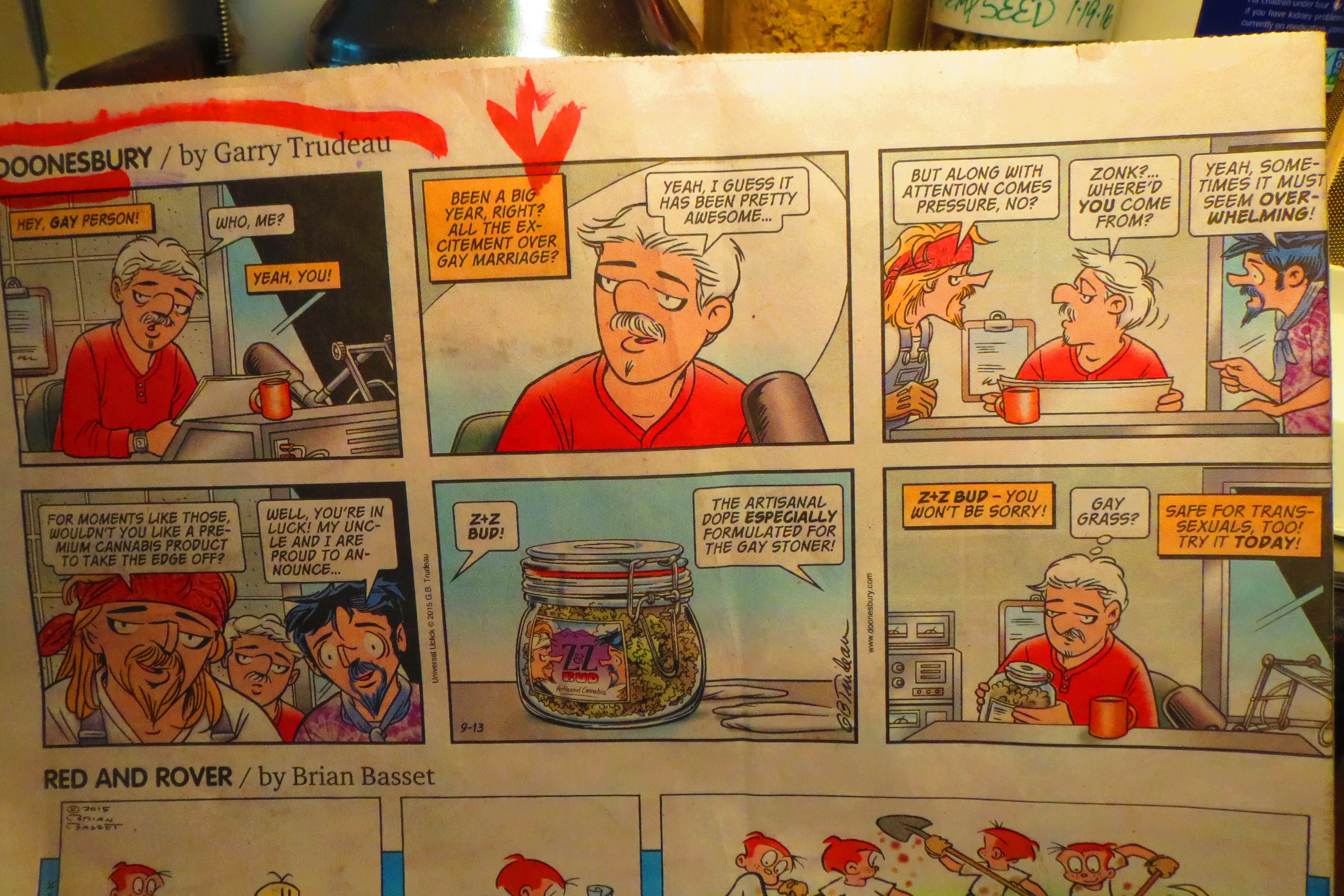The image captures a satirical Doonesbury comic strip by Garry Trudeau. The strip is divided into two rows of three panels each, presented on an old newspaper with a white background. In the upper left corner of the strip, the title "Doonesbury" and "by Garry Trudeau" are highlighted with a red marker and an arrow pointing at it. 

In the first panel, an older gentleman with white hair, a gray mustache, and a red shirt reacts to someone shouting, "Hey, gay person!" He responds with, "Who, me?" to which the voice confirms, "Yeah, you." In the second panel, the voice says, "Been a big year, right? All the excitement over gay marriage," and the man agrees, "Yeah, I guess it has been pretty awesome."

The third panel introduces two new characters: one with blonde hair and a red bandana, the other with black hair. The man with the bandana comments, "But along with attention comes pressure, no?" Confused, the older gentleman asks, "Zonk, where'd you come from?" The man with black hair adds, "Yeah, sometimes it must seem overwhelming."

The fourth panel offers a solution, as the man with the bandana proposes, "For moments like those, wouldn't you like a premium cannabis product to take the edge off?" His companion elaborates, "Well, you're in luck. My uncle and I are proud to announce," leading to the fifth panel, which showcases a jar labeled "Z+Z Bud." The product is described as "The artisanal dope specially formulated for the gay stoner."

In the final panel, the elderly man in the red shirt holds the jar, looking puzzled, as voices in the background chant, "Z+Z Bud, you won't be sorry. Safe for transsexuals too, try it today." He muses, "Gay grass," while examining the cannabis jar. Below the comic, a snippet of another strip titled "Red and Rover by Brian Bassett" is partially visible.